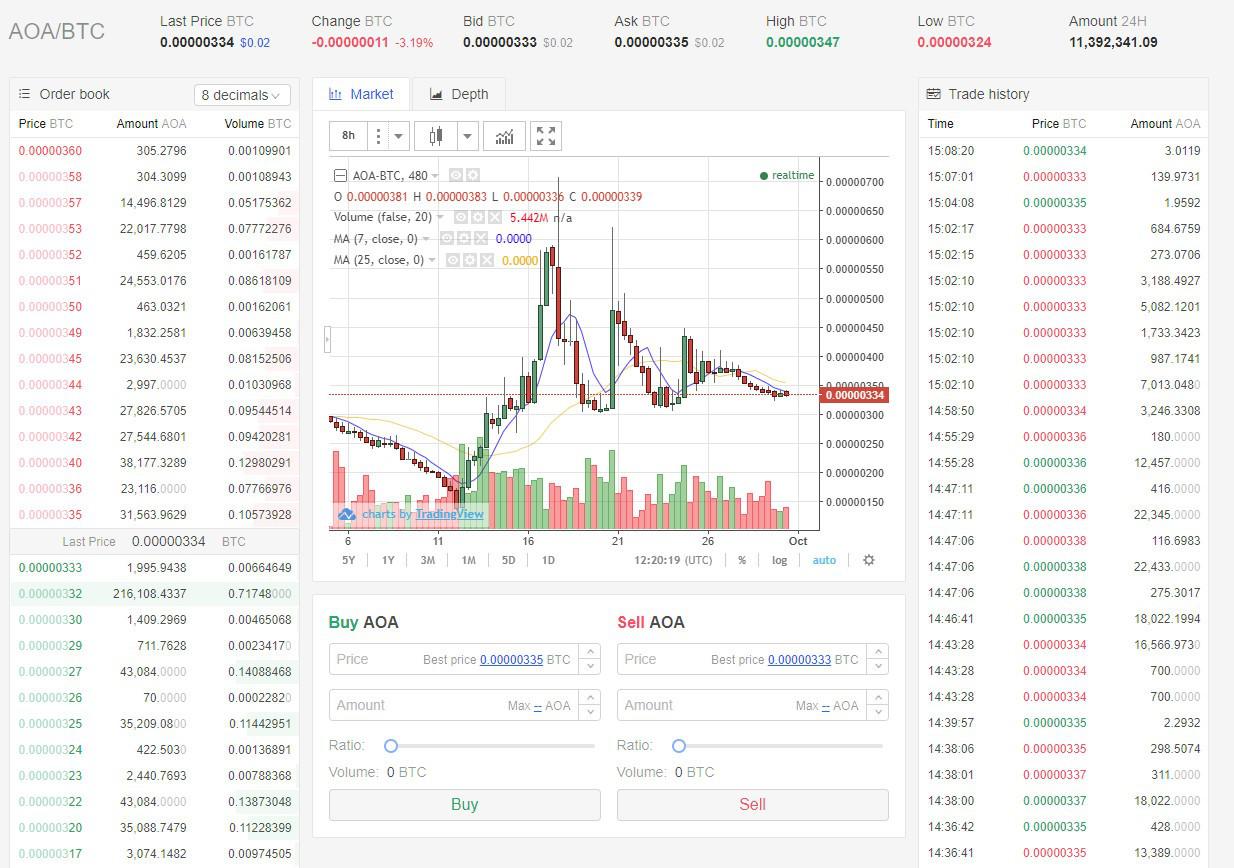The image appears to be a screenshot of a cryptocurrency trading interface, likely from an app, website, or program. The main focus is a chart monitoring Bitcoin trading pairs, specifically labeled as AOA/BTC. The background of the interface is predominantly light gray, with dark gray and blue accents for text.

Starting at the top left corner, the section provides key metrics:
- "Last Price BTC": The value here is a very small number, represented with several leading zeros (0.00000034 BTC) followed by a blue-highlighted value of 0.02.
- "Change BTC": This metric shows a negative value, with a minute change indicated (approximately -0.000000011 BTC) in red, complemented by a percentage change of -3.19%.

Further to the right, additional details are provided in black:
- "Bid BTC": The bid price is listed as 0.0000000333 BTC and a recurring figure of 0.02 is noted repeatedly across several columns.

The lower portion of the interface displays two distinct charts:
- On the left side, there's the "Order Book," showing the price, amount, and volume for Bitcoin buy and sell orders.
- On the right side, the "Trade History" lists recent transactions with corresponding Bitcoin prices, amounts, and total volumes traded.

The layout and color coding (red for negative values, blue for specific highlights) help users quickly interpret the trading data and market trends.